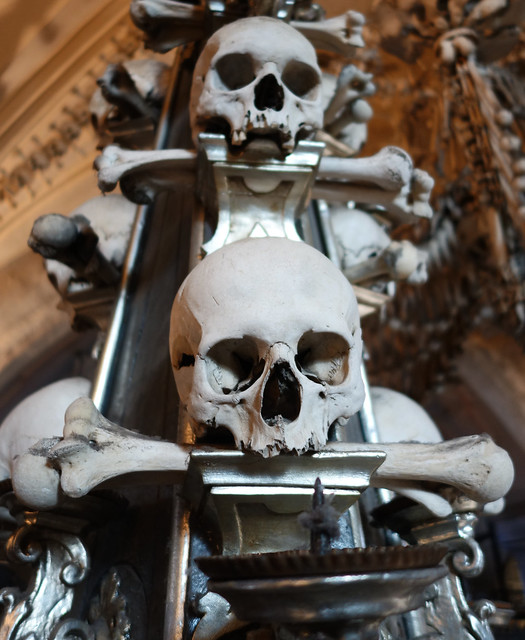The image features two prominent white human skulls, each distinctly positioned one atop the other. Both skulls exhibit significant metallic elements within their mouths, characterized by large bones protruding from either end of the metal. Their eyes and nasal cavities are notably absent, enhancing the skeletal effect. Below the lower skull, there is an object resembling a brush with a metal back and a pointed protrusion. Surrounding the central figures are various metallic elements, creating an ornate appearance, with a tannish, blurry background and noticeable black objects to the left. The scene is framed with additional silver objects at the bottom left, and the image appears to be cropped on all sides.